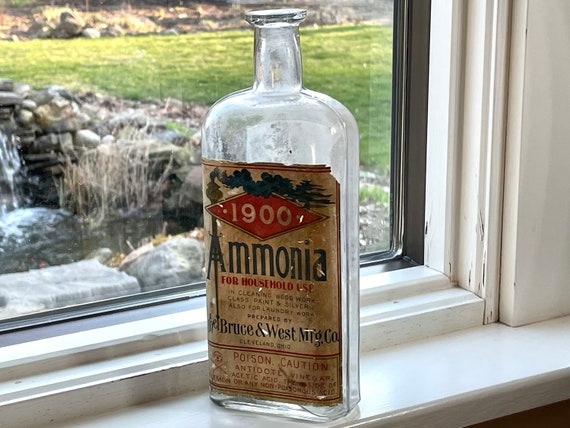A vintage, dusty clear glass bottle labeled "1900" in a prominent red diamond is carefully placed on a slightly worn, white wooden window sill in the bottom right-hand corner. The bottle, titled slightly to the left in contrast to the window's slight tilt to the right, boasts a brownish, weathered label with faded red and blue accents. The label reads "ammonia" in blue capital letters, followed by text indicating its use for household cleaning, specifically for paint and silver, and it's manufactured by Bruce and West Manufacturing Company. At the very bottom of the label, a red caution notice with a skull and crossbones prominently warns of poison. The clear, empty bottle stands as a silent relic against the backdrop of a well-lit, serene yard with vibrant green grass and a rocky, multi-leveled waterfall, the scene framed perfectly within the window.